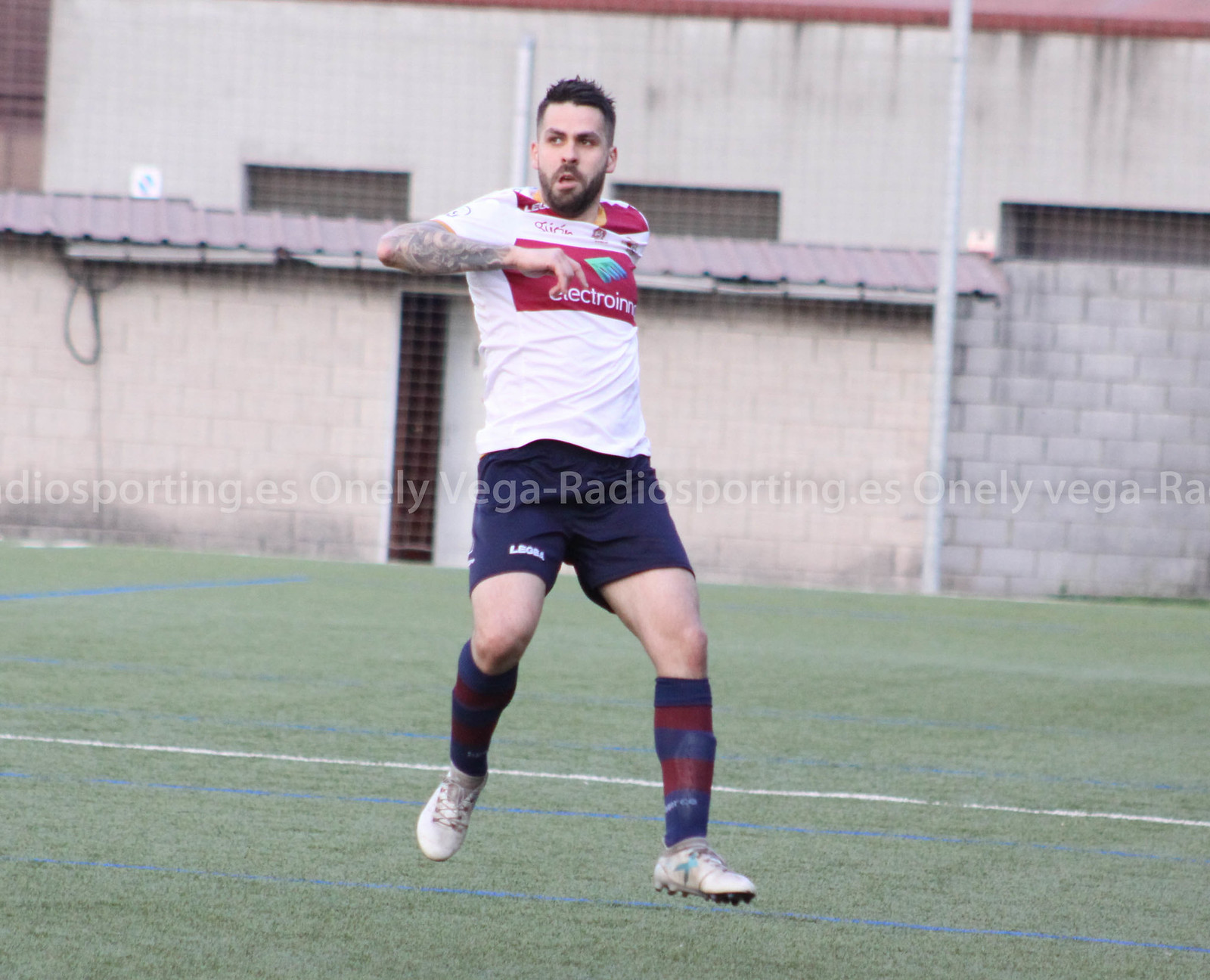This wide rectangular photograph captures a solitary soccer player positioned centrally on a grayish green turf. The field, occupying the lower half of the image, features thin blue and white painted lines and appears to tilt slightly downwards towards the right edge. The edge of the field is bordered by an off-white to gray brick wall with a reddish metal roof atop. Beyond this structure, a taller, gray building with caged windows can be seen, giving the background an industrial look.

The soccer player, a bearded man with fair skin and tattoos on his right arm, is captured mid-motion with his left foot barely touching the ground's tip. He wears a primarily white t-shirt with a red logo or block design at the chest, navy shorts with faint white text, and white athletic shoes with cleats. His right arm is positioned against his chest, and he seems to be looking off to his left. The field appears empty, with no other players or sky visible, and across the image's center is a transparent, repeating watermark text that reads "O-N-E-L-Y P-E-G-A radio sporting dot E-S". The scene is set outdoors in what seems to be daylight.